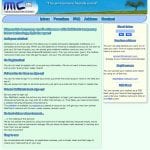This is a screenshot of a very blurry webpage, making the text and finer details difficult to discern. At the top, there is a banner featuring the letters "MC" on the left side, with some indiscernible gray writing beneath them. To the right of the banner, there appears to be an image depicting blue water, green grass, and a solitary tree. Below the banner, the webpage has a navigation bar with five tabs. The tabs are presented on a light blue background with dark blue lettering, though the text itself is unreadable due to the blurriness.

Further down, there is a section with a pale green background that includes a title written in blue lettering. This section is divided into six subsections, each containing a paragraph or a few sentences of text. To the right of this section, there is a smaller area with a pale yellow background featuring some bold and light blue text. This area also includes two call-to-action buttons.

Finally, the bottom part of the webpage is divided into three sections, each containing a paragraph or a few sentences of text. Overall, while the layout and colors of the webpage are somewhat distinguishable, the actual content and specific details remain unclear due to the poor image quality.